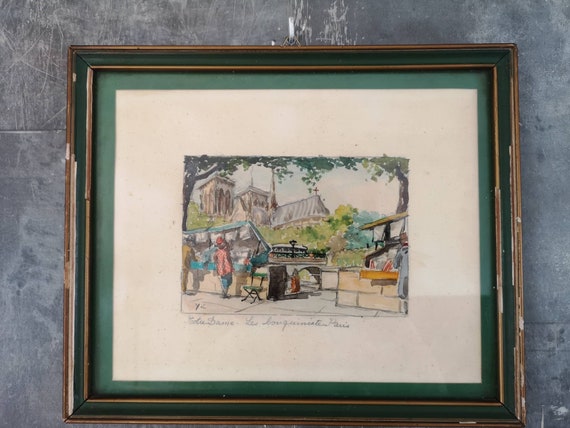The image depicts a photorealistic watercolor painting housed in an ornate frame featuring green with gold trimmings. The frame sits against a darker, concrete-like wall that appears scratched and uneven. The painting itself is presented on canvas-colored paper surrounded by a green mat with a white inner border. The scene captures a quaint European-style town with old stone buildings, including a church visible in the background. In front of the church, a small wooded area extends toward the middle ground. The bottom third of the painting is bustling with people shopping at market stalls and stands situated in front of what looks like a bridge or a canal walkway. All the shoppers are seen from behind, engaged in their activities under a canopy of trees. The scene signifies a clear, daytime atmosphere with a blue sky and some clouds. Additionally, there is some text below the image, though the letters are too small to discern.